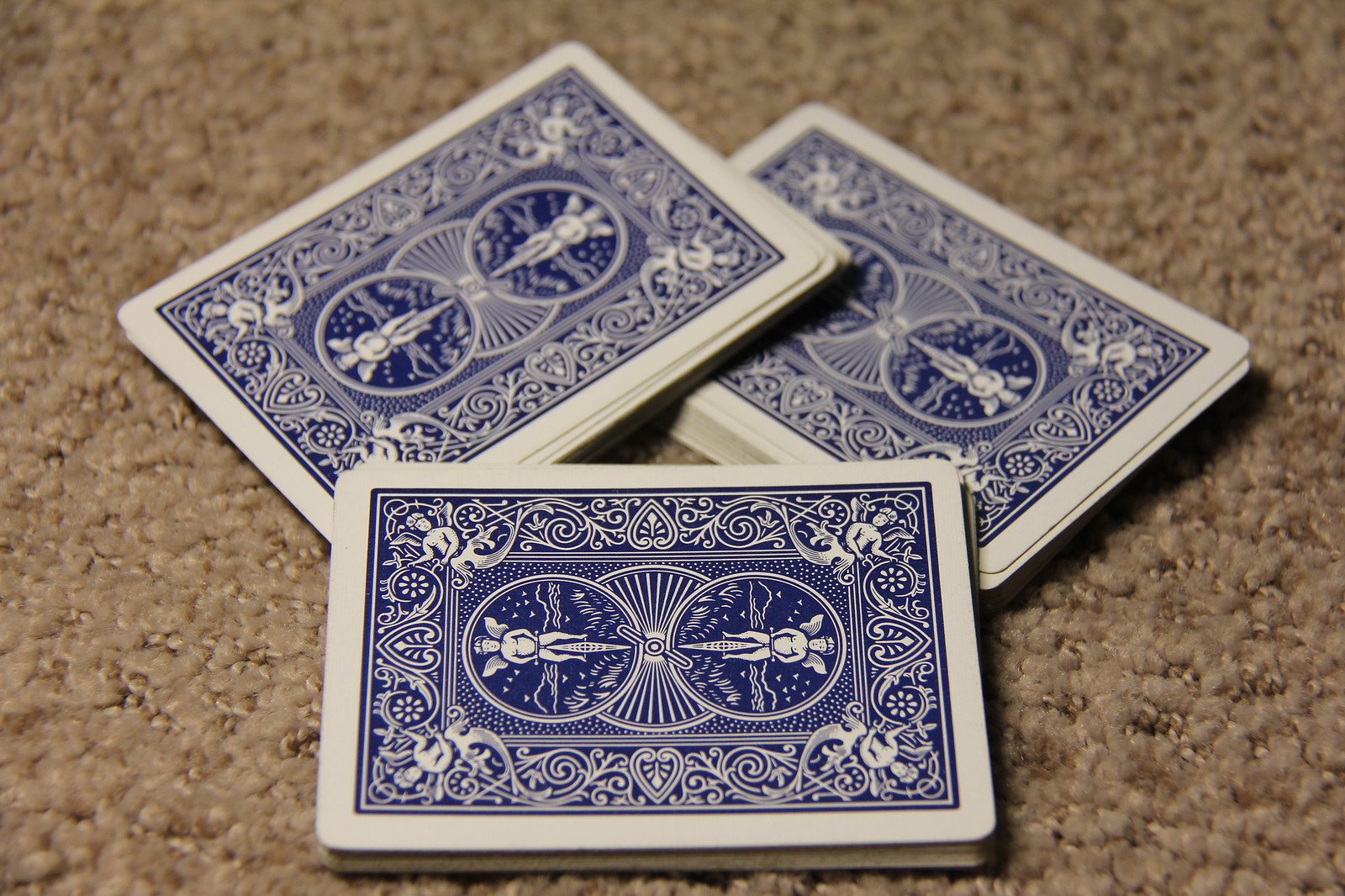This is a photograph showcasing three small stacks of standard blue playing cards meticulously arranged to form a triangular structure. The first stack is positioned on the left at a 90-degree angle, leaning against the second stack. This second stack, in turn, also rests partially on the beige carpet. The third stack lies horizontally in front of these two, with one long edge on the carpet and the other supported by the first two stacks. The arrangement results in an intricate, balanced triangular shape. The blue cards feature a symmetrical design, with an illustration of a fairy person that appears mirrored on either side if the card were folded down the middle. The stacks vary in depth, containing approximately 20, 16, and 8 cards, respectively, and add a detailed and slightly whimsical element to the composition against the soft, neutral backdrop of the carpet.